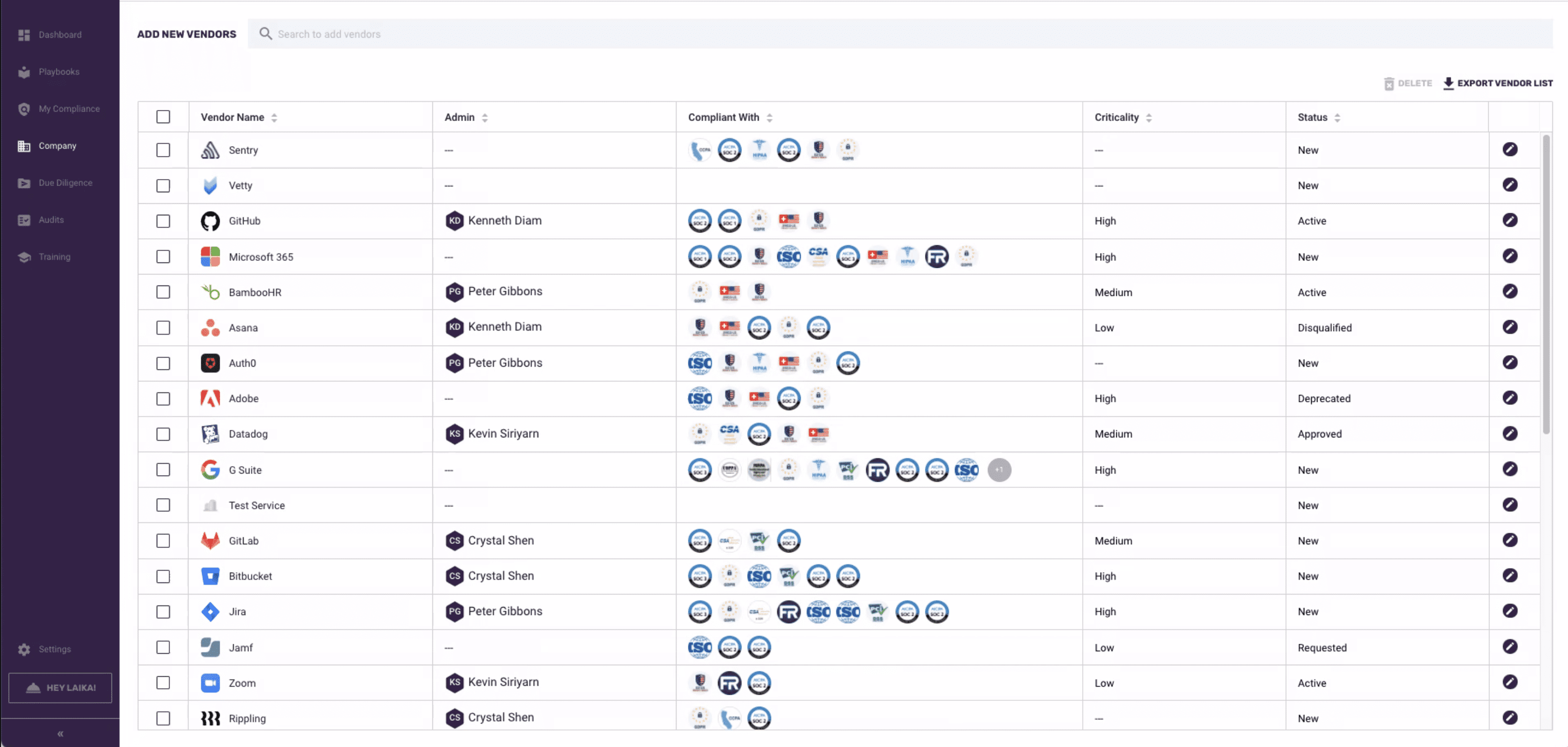The left side of the image features a purple bar with text indicating "New Vendors." Below this bar is a section equipped with a magnifying glass icon for searching vendor names, showcasing a diverse list of vendors.

On the right side of the image, there are options for "Delete," "Export," and "Render." The navigation menu on the left includes the following sections: Dashboard, Playbooks, My Client, Company, Due Diligence, Audits, Training, and Settings. Additionally, there are listed vendor names including Helica, Sentry, Microsoft 365, Asana, Acero, Adobe, Datadog, G Suite, Test Service, GitLab, Zoom, and Rippling.

Administrator details are displayed, listing Kenneth Diem, Peter Gibbons, Kevin Sirian, and Crystal Chen. Each administrator appears multiple times, indicating perhaps their association with various tasks or departments.

There is a compliance section featuring symbols that denote different levels of criticality, categorized as High, Medium, and Low. 

At the top of the image, vendor status labels include “New,” “Active,” “Disqualified,” “Deprecated,” “Approved,” and “Requested,” with varying status distributions across the vendors.